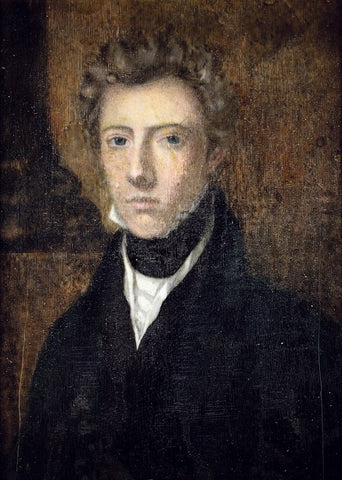The image depicts an old painting, possibly from the Renaissance period, portraying a stoic male figure with dark eyes staring straight ahead. The background is a textured, grainy brown color. The individual, who presents a blend of traditionally masculine attire and slightly feminine facial features, has medium brown, wavy hair pushed back, revealing a slight widow's peak. He wears a black jacket over a white undershirt, which is completely closed, concealing any additional details of the shirt. Around his neck is a black fabric that could be a handkerchief or collar, adding a touch of formality to his appearance. The painting captures a timeless, contemplative expression on the man's face, framed by the simplicity and depth of the dark background.